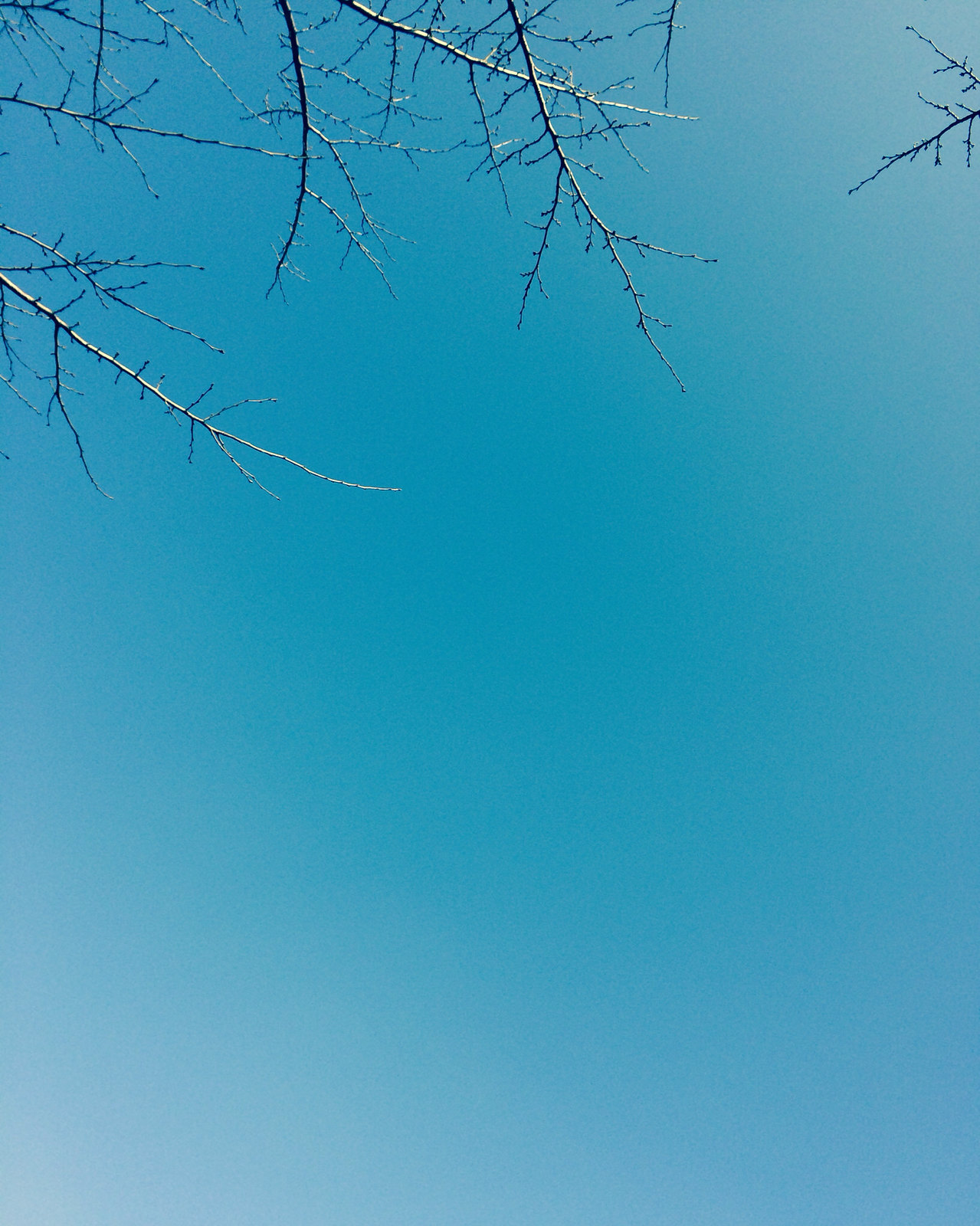The photograph captures a person looking directly up at the sky during a bright daytime. The sky, a light blue color, dominates the background, with the edges of the photograph appearing lighter and whiter due to the lighting. The top of the image is adorned with barren tree branches—three in the top middle and top left, and two in the top right—each branch having multiple smaller branches extending from them. No clouds or foliage are present, making the stark grayish-brown branches a striking contrast against the serene blue sky.